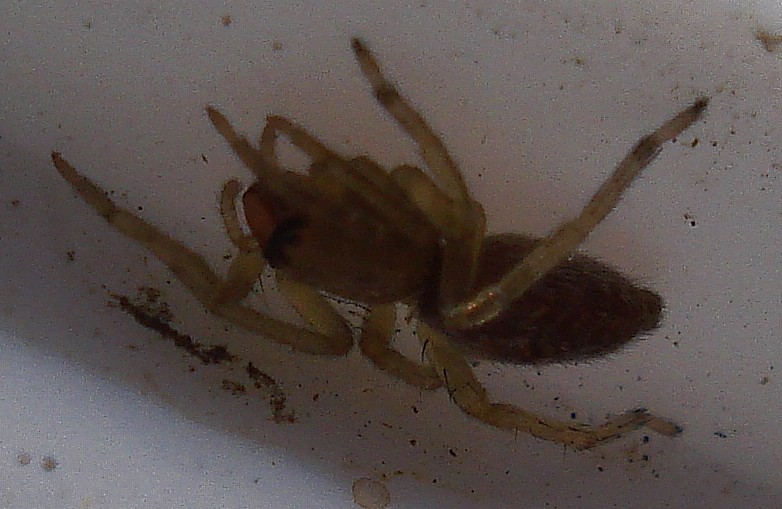The image is an extreme close-up photograph of a spider clinging to a dirty white surface, covered in various gray specks, dirt, and detritus. The spider is a brownish color with semi-translucent tan legs, which allow visibility through its entire body and front pincers. The body features a darker brown hue with black circles where its eyes are located and showcases a darker brown stripe pattern on its abdomen. The spider, which appears to have eight segmented legs, is facing toward the top left corner of the image and seems to be upside down. The background has a notable contrast, with the top left-hand corner being lighter compared to the dark and shadowed areas, highlighting the speckled and dirty condition of the surface.